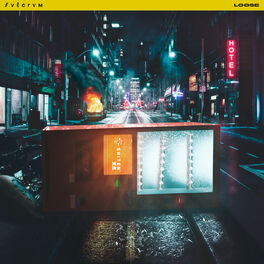The photograph captures a deserted city street at night, freshly glistening from recent rain. Dominating the foreground is a toppled red vending machine or cabinet, emitting a blue glow from a screen that displays three gray posts with black holes. An orange panel with white circles is also visible on the device. The background reveals a vanishing point perspective of a city street lined with streetlights on both sides forming an upside-down 'V', leading to a series of indistinct establishments with neon and LED signage. To the right, a bright neon sign reads "Hotel" in white letters against a red backdrop. Above the scene, a yellow border runs across the top of the photograph, inscribed on the left with "S-V-T-E-R-V-M" and on the right with "L-O-O," rendered in unconventional lettering. A distant skyscraper looms at the end of the street, adding to the sense of urban isolation. The street appears eerily quiet, with no people in sight and an atmosphere of desolation pervading the scene.